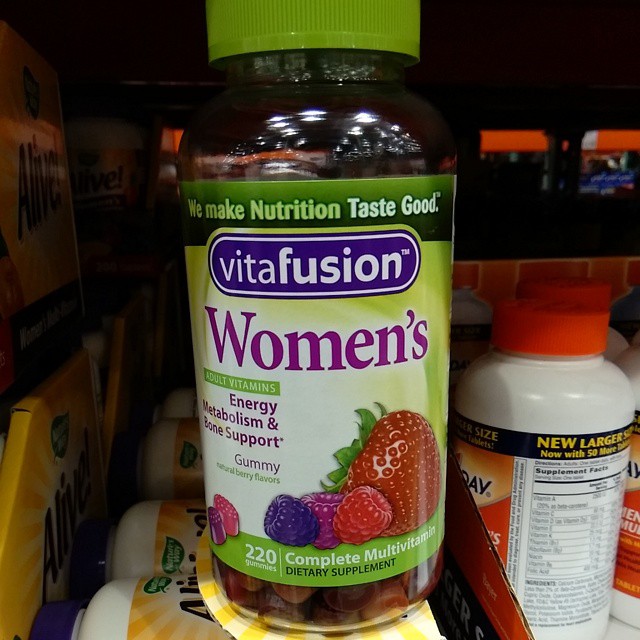This image captures a bottle of VitaFusion Women's Adult Vitamins—a dietary supplement designed to support energy metabolism and bone health. The bottle prominently displays the product's name, "VitaFusion Women's Adult Vitamins Energy Metabolism and Bone Support," and highlights its key features. The bottle contains 220 natural berry-flavored gummies, visible through the clear bottom section of the container. The label, which covers approximately three-quarters of the bottle, features a vibrant color scheme including green, purple, red, and blue. The text on the label is primarily green and purple, matching the green cap. The visually appealing design underscores the product's dedication to delivering a delicious and healthy multivitamin option.